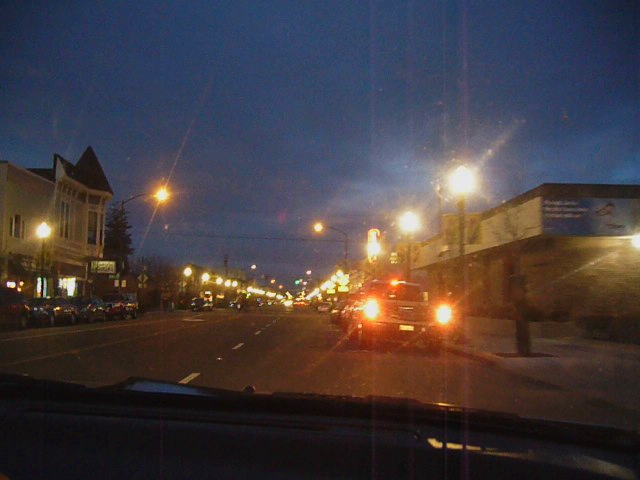This nighttime photograph captures a bustling four-lane city street, viewed from inside a car looking through the front windshield. The dark blue sky, dotted with clouds, casts a serene backdrop, while the street is illuminated by bright, glare-inducing streetlights lining both sidewalks. Cars are parked on either side, including one on the right facing the wrong direction, its brake lights glowing as if it is just parking or preparing to leave. Oncoming traffic is visible, with a vehicle's red front headlights standing out. Buildings of up to two stories and clearly visible footpaths add to the urban scenery, and the double yellow lines and white dashed lines mark traffic regulations on the road.